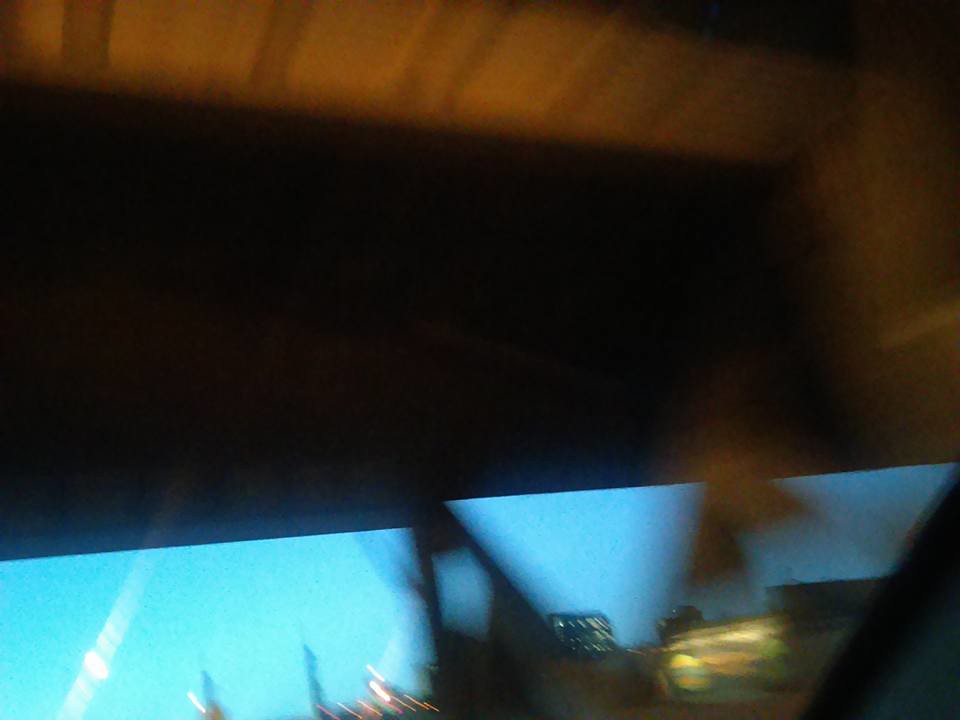This image is a very blurry photograph, making it difficult to definitively identify the subject. The top section features a sort of orange-tan hue with darker brown areas below it. Towards the center-top, there's a hint of black horizontal color, possibly indicating shadows or the edge of a structure. Below this darker section, a sky blue area emerges, potentially depicting light from a window or a brightly lit outdoor scene.

On the bottom right corner, there are splashes of more vibrant hues—red, yellow, green, pink—suggestive of lights on buildings. Additionally, there is a diagonal black line intersecting the lower part of the image, adding to the distortion. The foreground is cluttered with various light patches and a distinct object in the center-bottom that seems to be triangular with an open center displaying blue colors, hinting at either a structure or a framing error.

Overall, motion blur or camera movement appears to have caused the entire image to be out of focus, giving the impression of a lighted building or cityscape viewed from a car or through a window, but ultimately leaving details too obscured to pinpoint accurately.